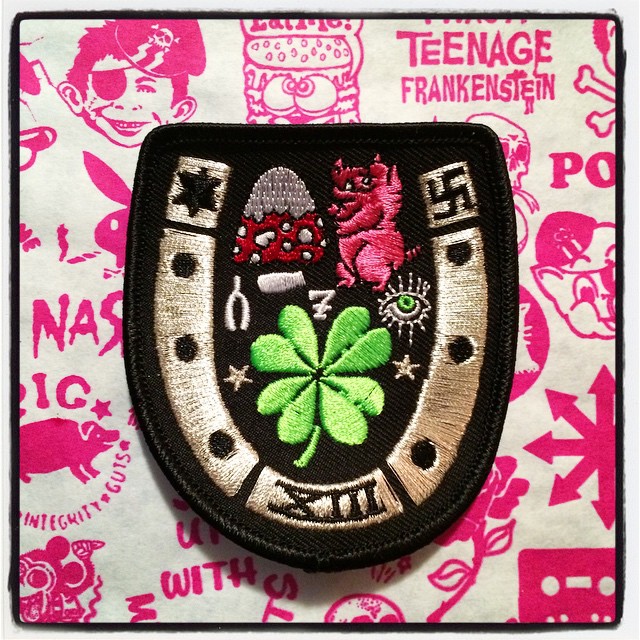The image showcases a detailed embroidered cloth patch centered against a vibrant graphic background. The background predominantly features pink and white, interspersed with cartoonish and symbol-laden drawings, including iconic images such as Alfred E. Neuman from Mad Magazine with a pirate cap and eyepatch, the Playboy bunny, and other American traditional tattoo art motifs. The patch itself, black in color, is shaped like a U with a flat top representing a silver horseshoe. On the left top of the horseshoe sits a star while the right top displays a swastika, and along its sides are black dots leading to the Roman numeral XIII at the bottom. Centered inside the horseshoe are eight green leaves resembling a clover, flanked by gold stars. Above this, a green eye with an East Asian pupil is depicted. Additional small images such as a mushroom, a wishbone, and a demonic figure are scattered across the patch. The phrase "Teenage Frankenstein" is prominently displayed in the upper right corner of the background, while other elements like a porky pig, flowers, and arrows further animate the lively patch.